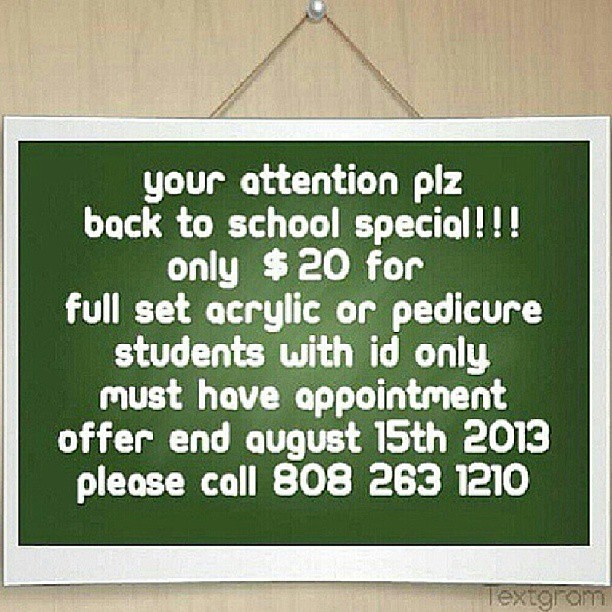The image features a digital advertisement for a special back-to-school sale, designed to look like a real-life sign hanging from a pearlish pin via twine. The sign has a green background with white text and an off-white border. It states, "YOUR ATTENTION PLEASE," followed by, "BACK TO SCHOOL SPECIAL," and "Only $20 for a full-set acrylic or pedicure. Students with ID only. Must have appointment. Offer ends August 15, 2013. Please call 808-263-1210." The entire text is in lowercase letters. The sign appears to be hanging against a pale wood-colored background, and in the bottom right corner of the image, the word "TEXTGRAM" is displayed in dark grey or brown text. The advertisement is outdated and its offer is no longer valid.